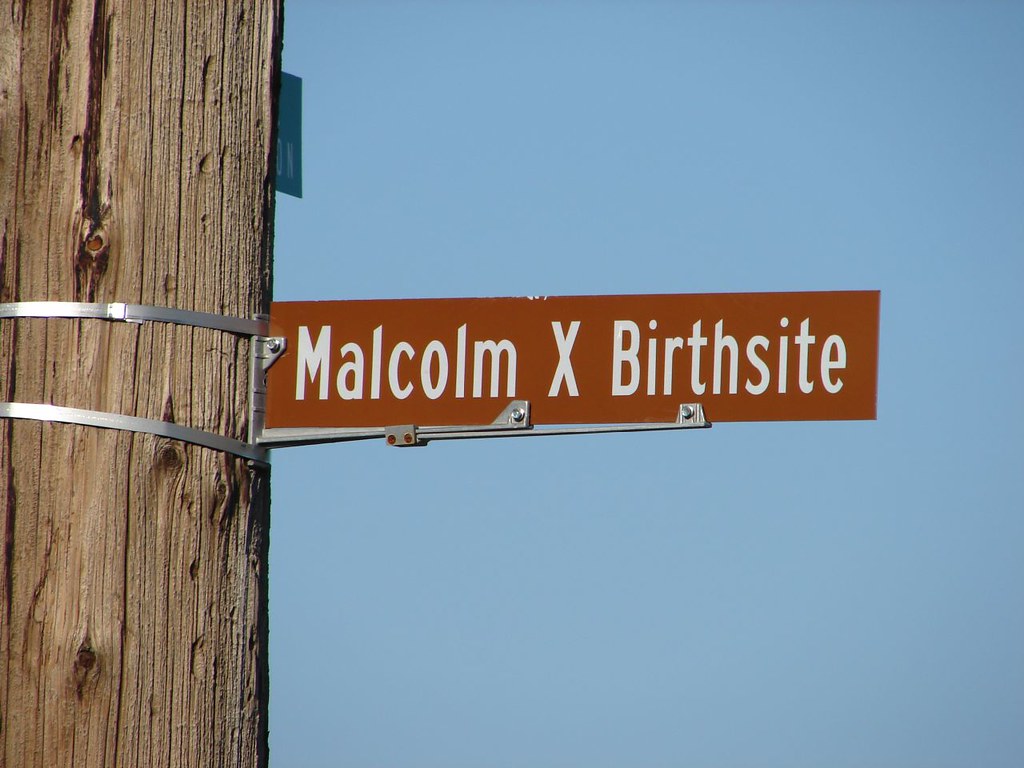This detailed image shows a close-up of a rectangular brown sign attached to a wooden telephone pole, held in place by two silver metal straps. The sign, prominently positioned in the center of the image, features white lettering that reads "Malcolm X Birth Site." The telephone pole, taking up about 25% of the left side of the image, extends vertically from top to bottom. In the background, a pale light blue sky stretches across the scene with no clouds visible, adding a serene backdrop. Part of another sign, possibly green or blue, is partially visible behind the telephone pole on the top left side.